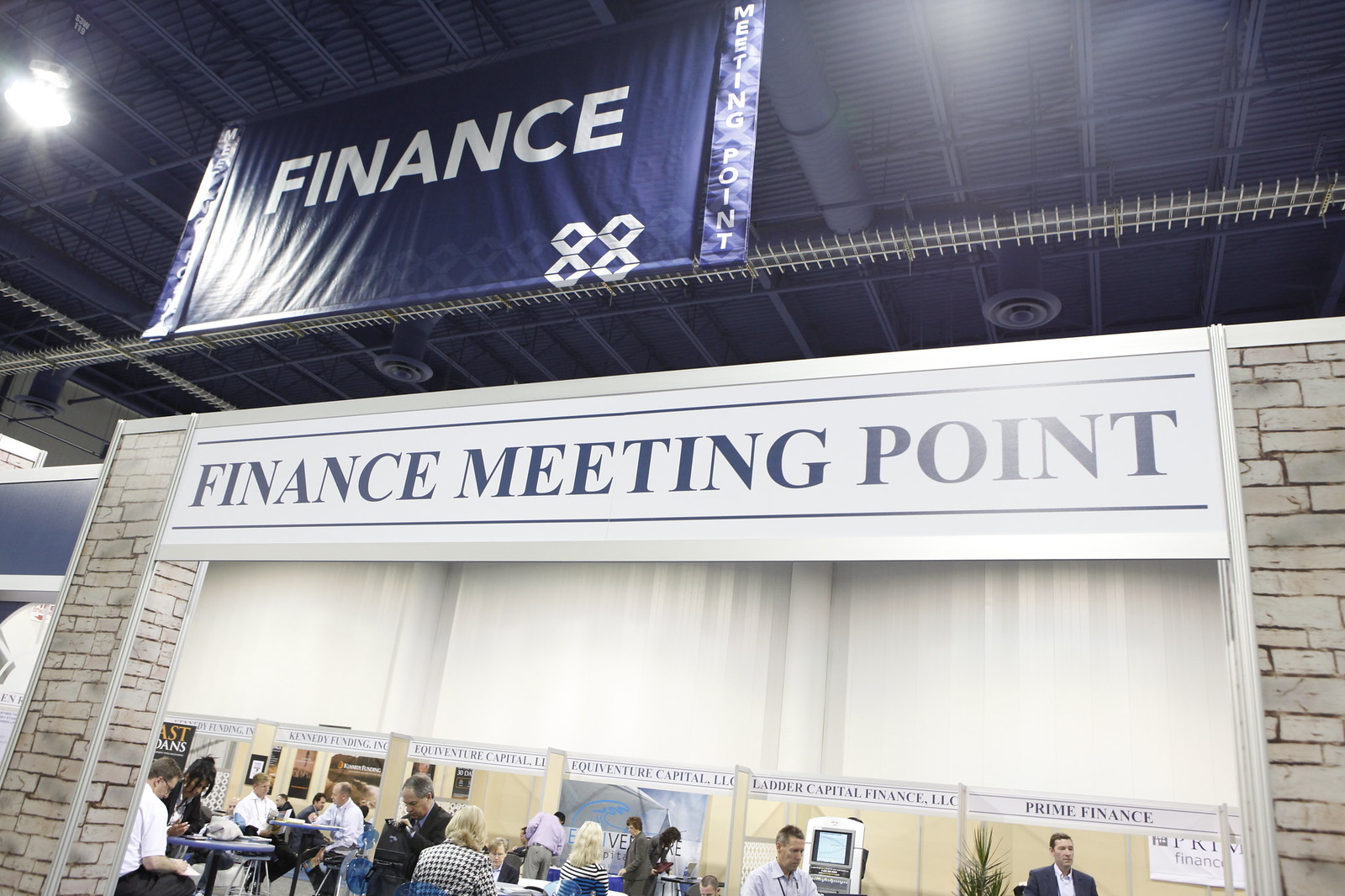The image showcases the bustling entrance of a large convention center dedicated to a financial expo. Dominating the top of the entrance is a prominent blue banner with "Finance" boldly printed in white. Just below, another sign reads "Finance Meeting Point," marking the focal area for attendees. This entrance is flanked by gray brick pillars, framing the scene. Inside the venue, professionals dressed in formal office attire mill about, engaging in discussions and presentations. Central to the setup is a small kiosk featuring multiple financial firms, including Kennedy Funding Inc, Equiventure Capitalist Inc, Ladder Capital Finance LLC, and Prime Finance—all gathered under one banner atop blue desks. The convention center's high blue metal rigging ceiling further emphasizes the scale of the event. In the background, a white-framed monitor provides additional information, contributing to the dynamic, information-rich environment of the financial expo.